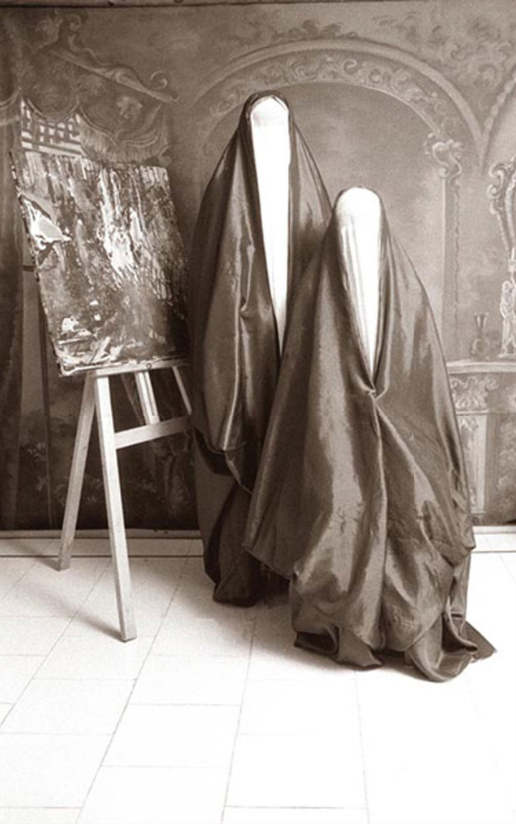In this black and white photograph likely taken years ago, we find a curious indoor scene that appears to be set in an art studio. Central to the composition are two figures dressed in striking outfits that fully obscure their identities. These figures, standing on a tile floor, are clad in long black robes that extend from their shoulders to beyond their feet. The robes feature a distinctive white, V-neck-like design that covers them from their heads down to their chests, giving them a somewhat uniform appearance that complicates any attempt to discern gender. 

Positioned directly beside these two anonymous individuals is an art easel bearing a painting, though its details remain indistinct due to the grayscale nature of the photograph. The backdrop consists of wallpaper adorned with elegant patterns, reminiscent of regal or classical designs, that enhance the already vintage aesthetic of the space. Despite the lack of visible text, the setting and the objects within hint at a creative and possibly historical context, blending the subjects seamlessly into their environment.